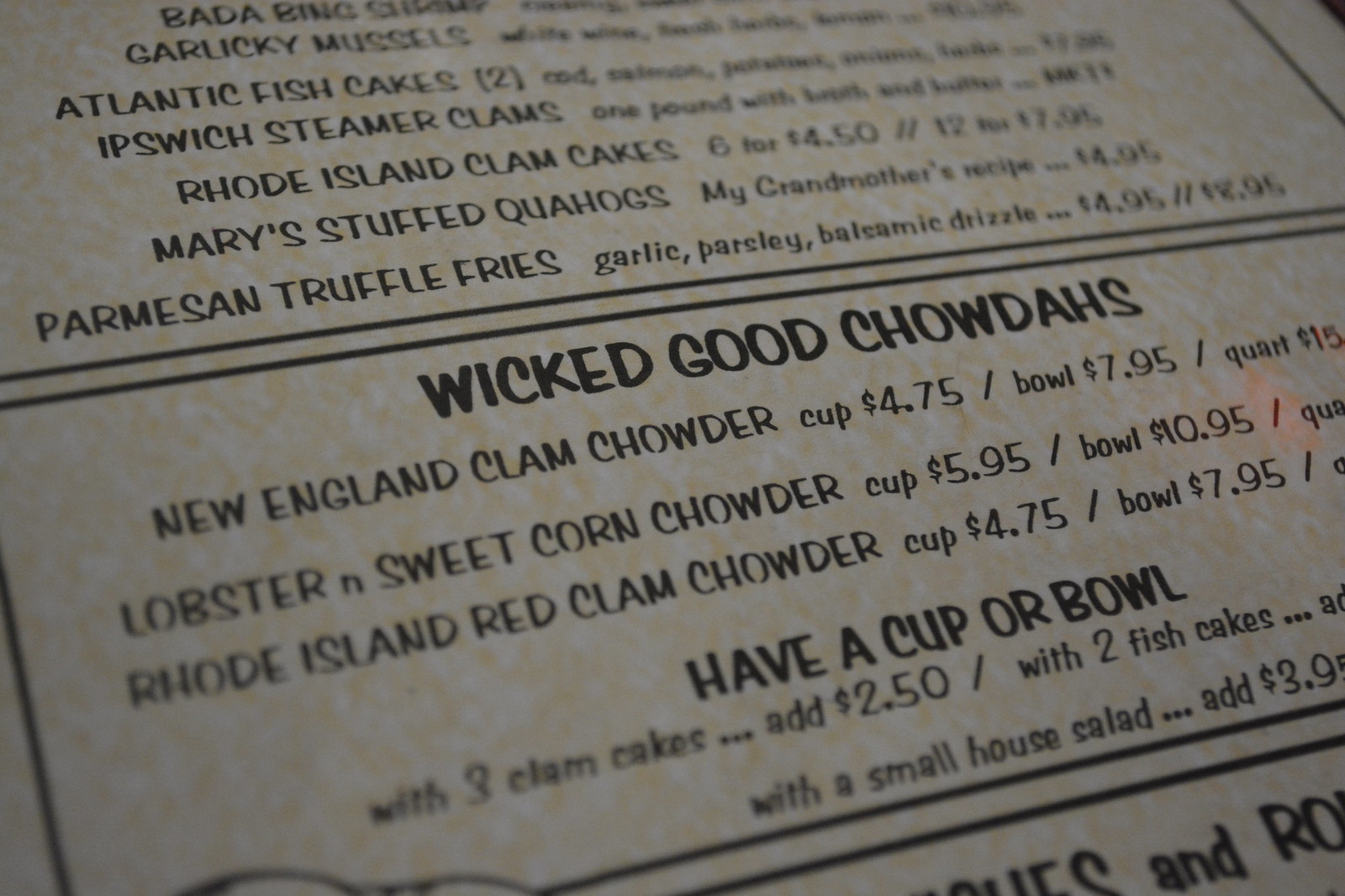In this photograph of a menu, the central focus is a section titled "Wicked Good Chowdahs," spelled humorously as C-H-O-W-D-A-H-S, in bold black letters. Below this heading, the menu details three chowder options:

1. **New England Clam Chowder**: 
   - Cup: $4.75
   - Bowl: $7.95
   - Quart: $15 (price partially cut off)

2. **Lobster and Sweet Corn Chowder**:
   - Cup: $5.95
   - Bowl: $10.95
   - Quart: (price cut off)

3. **Rhode Island Red Clam Chowder**:
   - Cup: $4.75
   - Bowl: $7.95

Additionally, customers can enhance their chowder experience by adding:
- Three clam cakes for an extra $2.50.
- Two fish cakes (price cut off).
- A small house salad for $3.95 (partially cut off).

The menu features distinct sections separated by black borders, with items somewhat out of focus at the top right and bottom left. Above the "Wicked Good" chowders, other offerings include:
- Parmesan Truffle Fries
- Mary Stuffed Quahogs
- Rhode Island Clam Cakes
- Ipswich Steamer Clams
- Atlanta Fish Cakes
- Garlicky Mussels